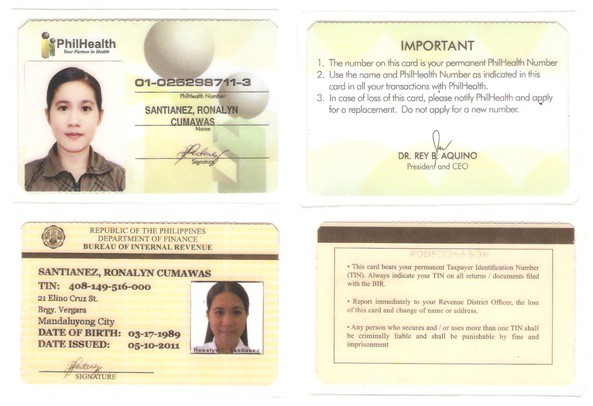This image displays two different identification cards for a woman from the Philippines, each shown from both the front and back, arranged in a 2x2 grid. The top-left card resembles a driver's license but is a PhilHealth card, featuring the PhilHealth logo on the top left, accompanied by two white circles on the right. Below the logo is a photograph of an Asian woman with short black hair, wearing a dark-colored shirt with a collar. Her PhilHealth identification number, name "Santianas, Rolanin" followed by "C-U-M-A-W-A-S," and her signature are listed beneath her photo. To the right, the back of this card contains important information about the cardholder. 

The bottom-left image is a second identification card from the Republic of the Philippines Department of Finance, Bureau of Internal Revenue. This card has a thin red bar across its top, under which the woman's name, date of birth (March 17, 1989), address, and signature are listed. This card also features a photo of the same woman, this time with long black hair, wearing a white shirt, and smiling. The corresponding back of this card, displayed on the bottom-right, includes further information, a magnetic strip, and additional details printed in black text. All cards are predominantly yellowish, with the PhilHealth card incorporating some green and white elements.